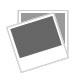This detailed and vertically aligned close-up photograph depicts a segment of a vintage calculator, possibly an old adding machine or a specialized keyboard. The device features a cream or beige-colored body with raised black keys that have white, all-caps text. Prominent keys visible in the image include a left arrow, an equal sign, a plus sign, a semicolon, a forward slash, an at sign, a return key, a question mark, a shift key, and a shift lock key. 

Towards the lower right corner, there are function-specific keys labeled "Charge," "On," "Off," and "Paper Feed," consistent with the calculator’s purpose. Above these, there is a small red light next to the label "Fast Charge." The photo also shows a dark, rectangular cut-out section at the top, which likely serves as an opening for inserting a paper roll, a common feature in old-style calculators with paper feeds. 

The overall tone of the machine is a blend of white or cream for the body and dark gray for the keys, with a concentrated black area around the charging slot. This intricate arrangement indicates the machine's specialized design and historical utility.